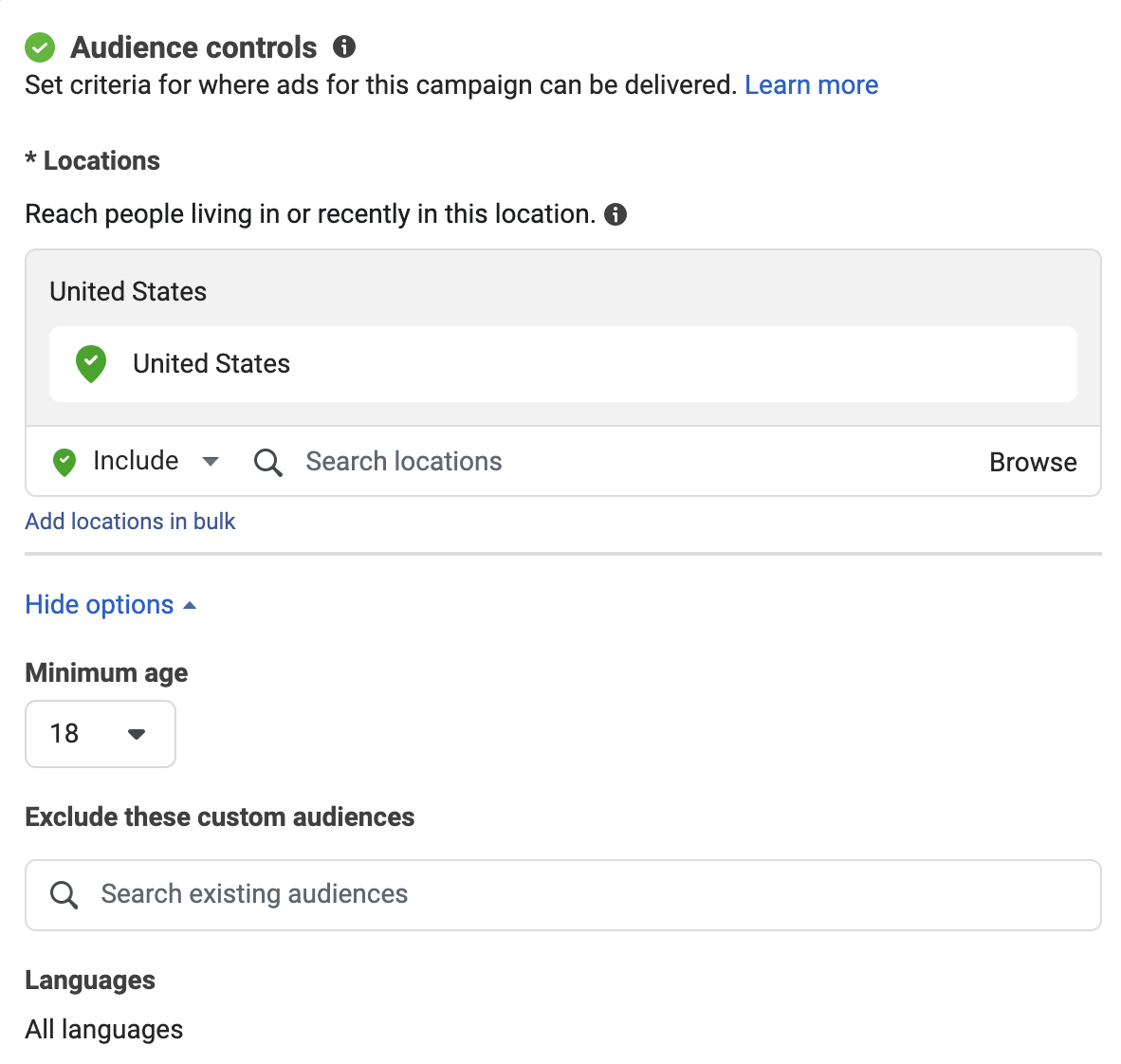A screenshot of a digital dashboard displays the "Audience Controls" section, used to set criteria for ad delivery parameters. This page appears to pertain to a campaign aimed at targeting specific audiences based on location, demographics, and other custom attributes. Central to the interface is the option to specify the audience's location, indicated by a green check mark confirming it's set for the United States. Additional options allow users to modify ad delivery based on people living in or recently in selected locations.

The layout features a clean white background interspersed with text in varying shades of black, ranging from bolded black titles to dark charcoal details. Accent colors include navy for "Ad Locations in Bulk" and a lighter blue for "Hide Locations," providing visual emphasis. Interactive elements such as setting minimum age (starting at 18), excluding custom audiences, and selecting languages (default set to 'All Languages') are prominently displayed. This comprehensive yet austere interface, devoid of any images, focuses entirely on enabling precise control over ad settings for a targeted campaign.